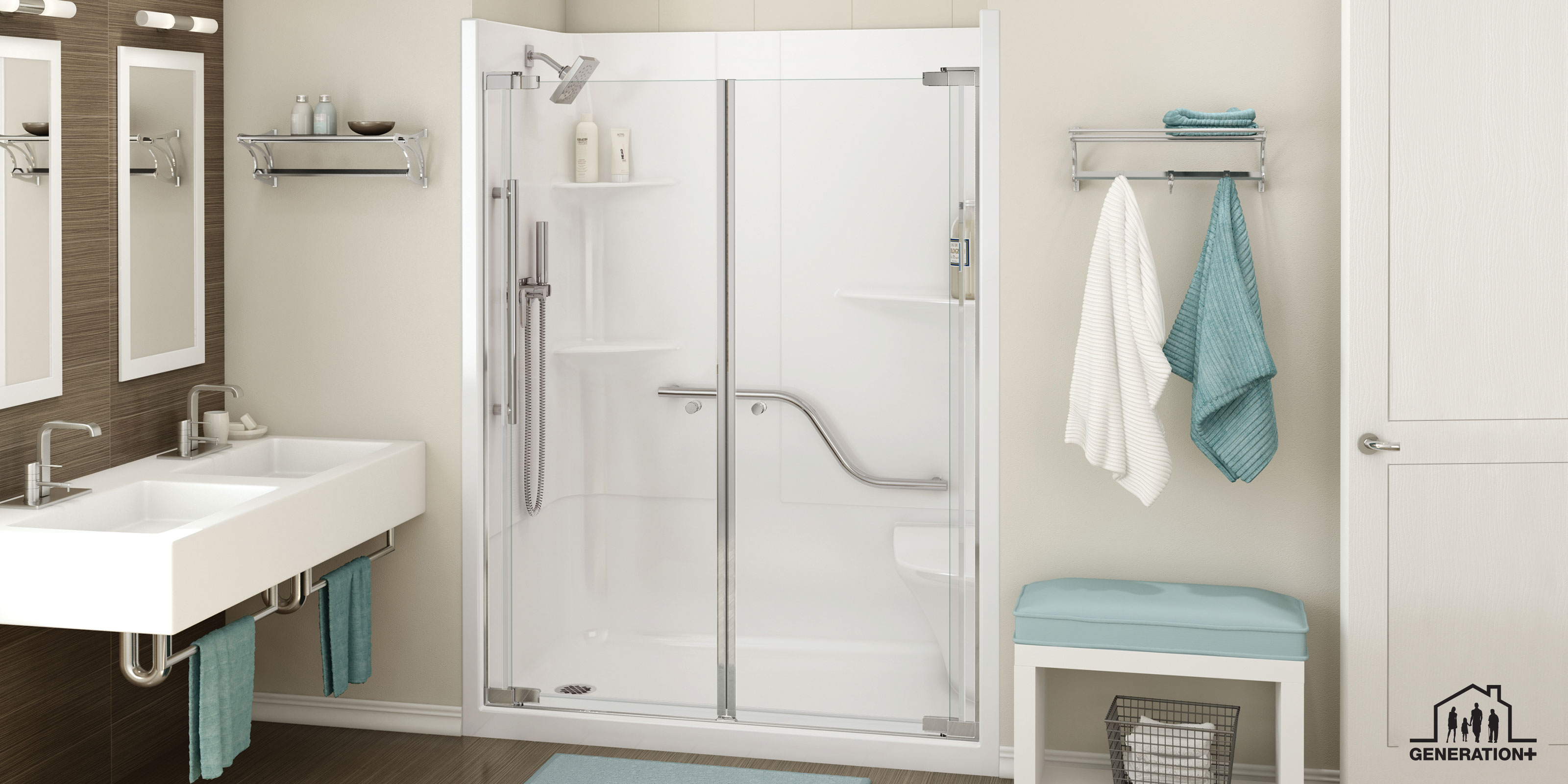The photograph captures a spacious and well-organized bathroom featuring a harmonious blend of light and dark tones. On the right side, a white door opens inward, inviting one into the bathroom. Adjacent to the door, a small shelf adorns the wall, holding a neatly folded turquoise towel on top, followed by a white towel and another turquoise towel hanging below on hooks. Beneath this shelving unit sits a turquoise bench, its cushion a delicate light blue hue, supported by white legs. 

A black mesh basket filled with meticulously folded white cloths enhances the bench's functionality and aesthetic. The shower, positioned to the left of the shelf, boasts a pristine white finish with sleek silver fixtures and clear doors. The interior of the shower is adorned with various shampoo bottles neatly arranged on the in-built shelving. 

The bathroom's walls are painted in soothing shades with a light beige covering the majority, contrasted by a darker brown accent wall facing the door. This darker wall features two rectangular mirrors with elegant white frames, each illuminated by overhead lights. Beneath the mirrors, twin white sinks with silver fixtures are linked together, complemented by silver bars that hold matching light blue towels.

To the left of the shower, an additional shelf holds a couple of bottles and a small dish, adding to the bathroom's organized charm. In the bottom right corner of the photograph, an outline of a house with people inside it serves as a logo for "Generation Plus," subtly integrated into the image.